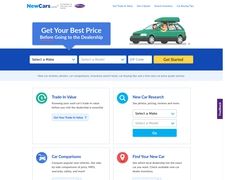The image depicts a partially legible website. At the top, there is a blue chat bubble positioned above a search bar with the text, “Get your best price. Better going to the deal, better going in the dealership,” or something similar. To the right of this, there is an image of a green hatchback car with a green canoe or paddle boat secured on top. Above this image, some text is present, though it is not clear. To the left, there is a heading where the word "new" is in a lighter blue color and "cars" is in a darker blue color.

Below the search bar, the webpage is divided into four sections, each containing an image thumbnail. The first thumbnail is green with a circular arrow pointing counterclockwise over it. Below this section, there is a blue icon with an indistinct white symbol inside. Moving to the right, the second thumbnail is light blue featuring a search icon. The third section presents a red location icon. The content and icons in these sections provide navigational or functional features of the website, though specific details are unclear.